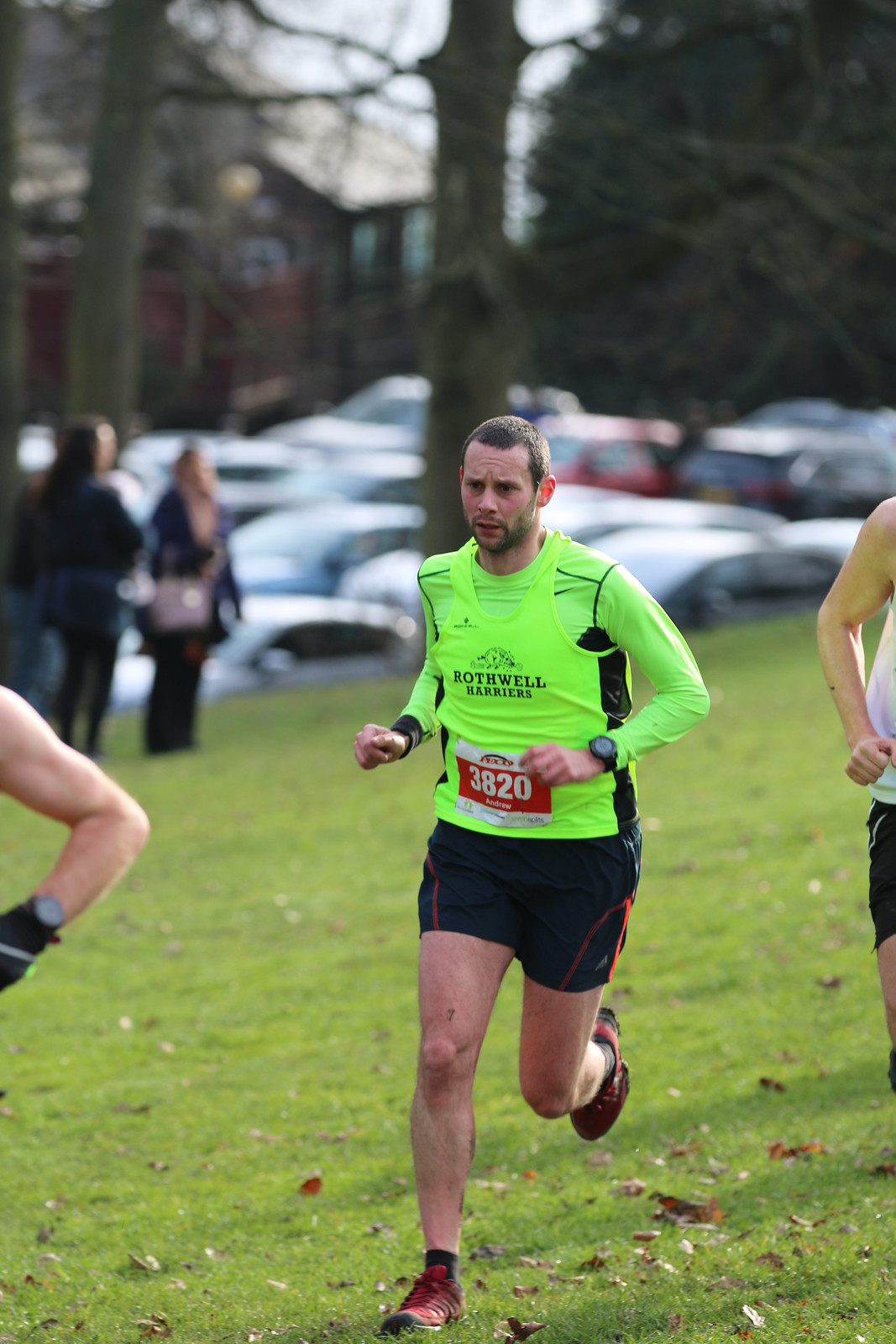The image captures a vibrant outdoor marathon scene centered around a male runner. The man is prominently positioned in the middle of the photograph, donning a neon yellow sleeveless tank top emblazoned with "Rothwell Harriers" and a large race number "3820" attached to its front. Beneath the tank top, he wears a matching neon yellow long-sleeve athletic shirt with black stripes along the seams and sides, paired with black training shorts that feature red or orange stripes. His footwear consists of red running shoes with black and red detailing, and he completes his gear with black ankle socks. 

The runner has short brown hair and a wristwatch on his left hand. Surrounding the central figure are the partially visible bodies of other runners on both sides, indicating a lively race atmosphere. The background reveals a grassy field scattered with spectators and parked cars, likely observing the marathon. Additionally, there is a brown building and multiple trees under a predominantly white sky, adding depth to the setting.